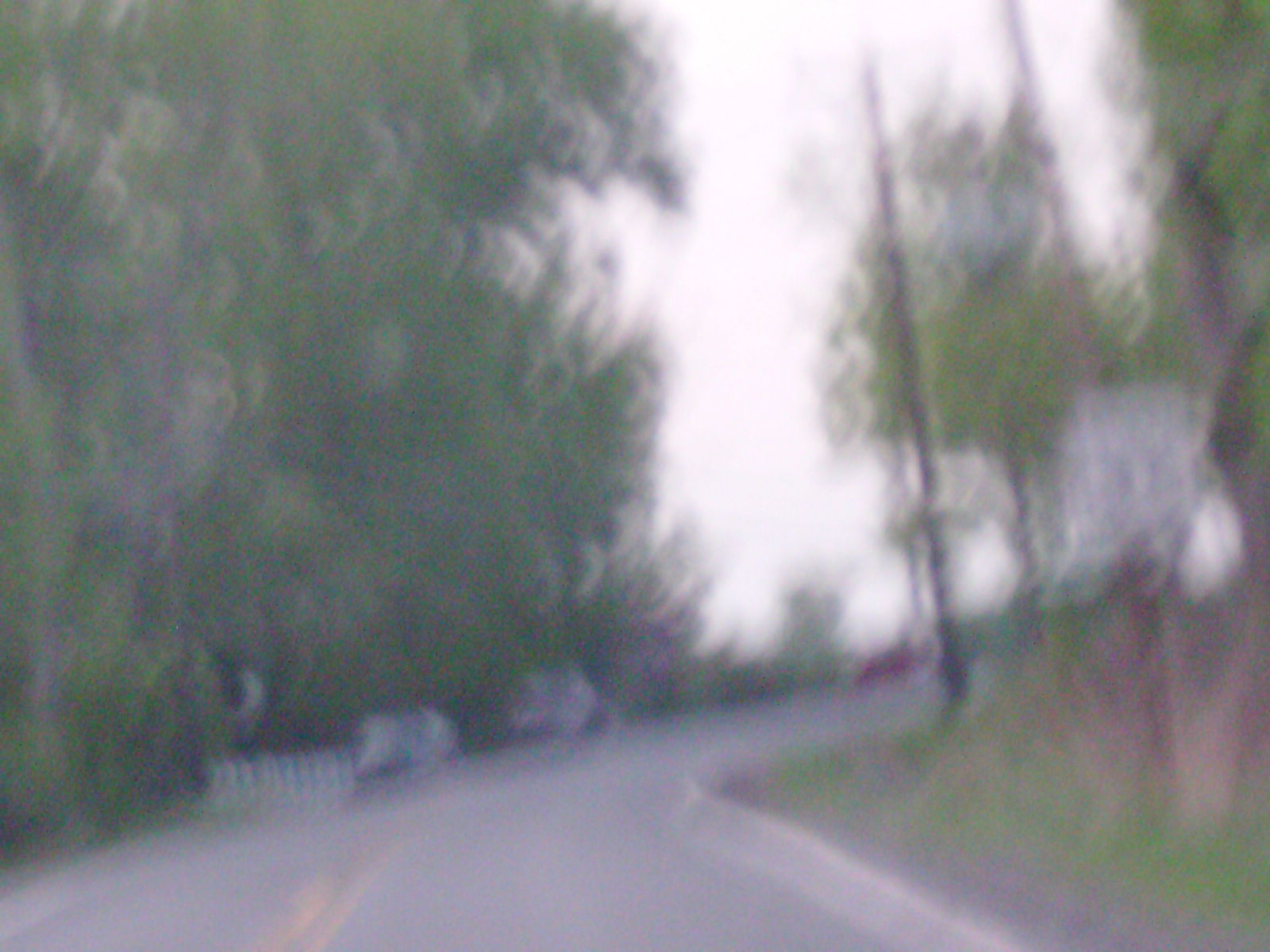This is a very blurry outdoor photo taken during the daytime, depicting a roadway that curves to the left. The road, which features a yellow stripe down the center, starts at the bottom right-hand corner and curves towards the left side of the image. On the right side of the road, there are several trees and some parked cars facing the camera, accompanied by a little white fence. The left side of the road is bordered by more large green trees and a white picket fence, extending from the bottom left corner to the middle of the picture. A 35 mph speed sign can also be vaguely seen on the left. There are power or telephone poles present, with one pole standing amidst tall weeds or grass to the right. The surroundings include patches of green grass near the curb and some areas of dirt. The sky appears cloudy with white and some darker clouds. The overall image is too indistinct for specific details due to its extreme blurriness.